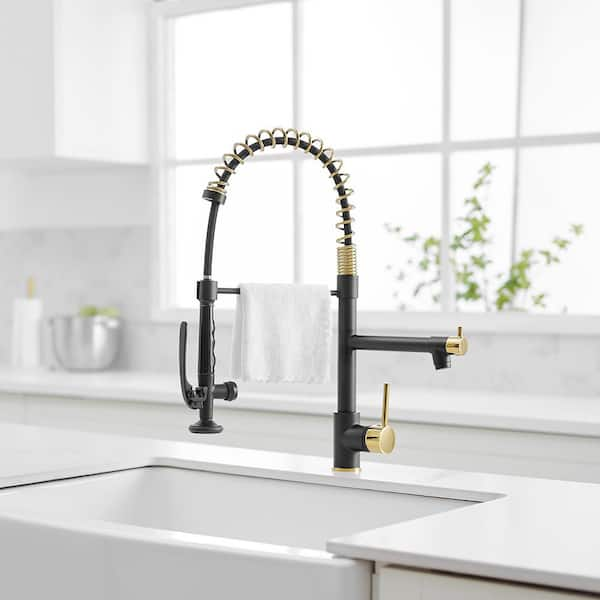This color photograph, in portrait orientation, showcases a sleek, modern kitchen setup with a distinctive kitchen faucet as the focal point. The faucet, a striking large upside-down U shape, is predominantly black and embellished with gold accent pieces. The end of the faucet features gold rods, and as it rises, the black material transitions into a gold spring housing a black tube, forming the arch. The black detachable spray head, integrated into the gold spiral, hangs above the pristine white recessed sink positioned centrally on the white countertop. The faucet, adorned with a brass round fitting and lever controls on the right, adds a touch of elegance and functionality.

Above the sink, a six-pane window fills the background, enhancing the space with natural light. The surrounding white cabinets and counter accentuate the faucet's bold design. On the left side of the counter, a roll of paper towels and a silver bowl with a green plant add practical and aesthetic elements to the scene. The setup is completed with a white towel hanging from the faucet, exemplifying the clean and minimalist aesthetic of the kitchen. This photograph epitomizes photographic representationalism and realism in product photography.